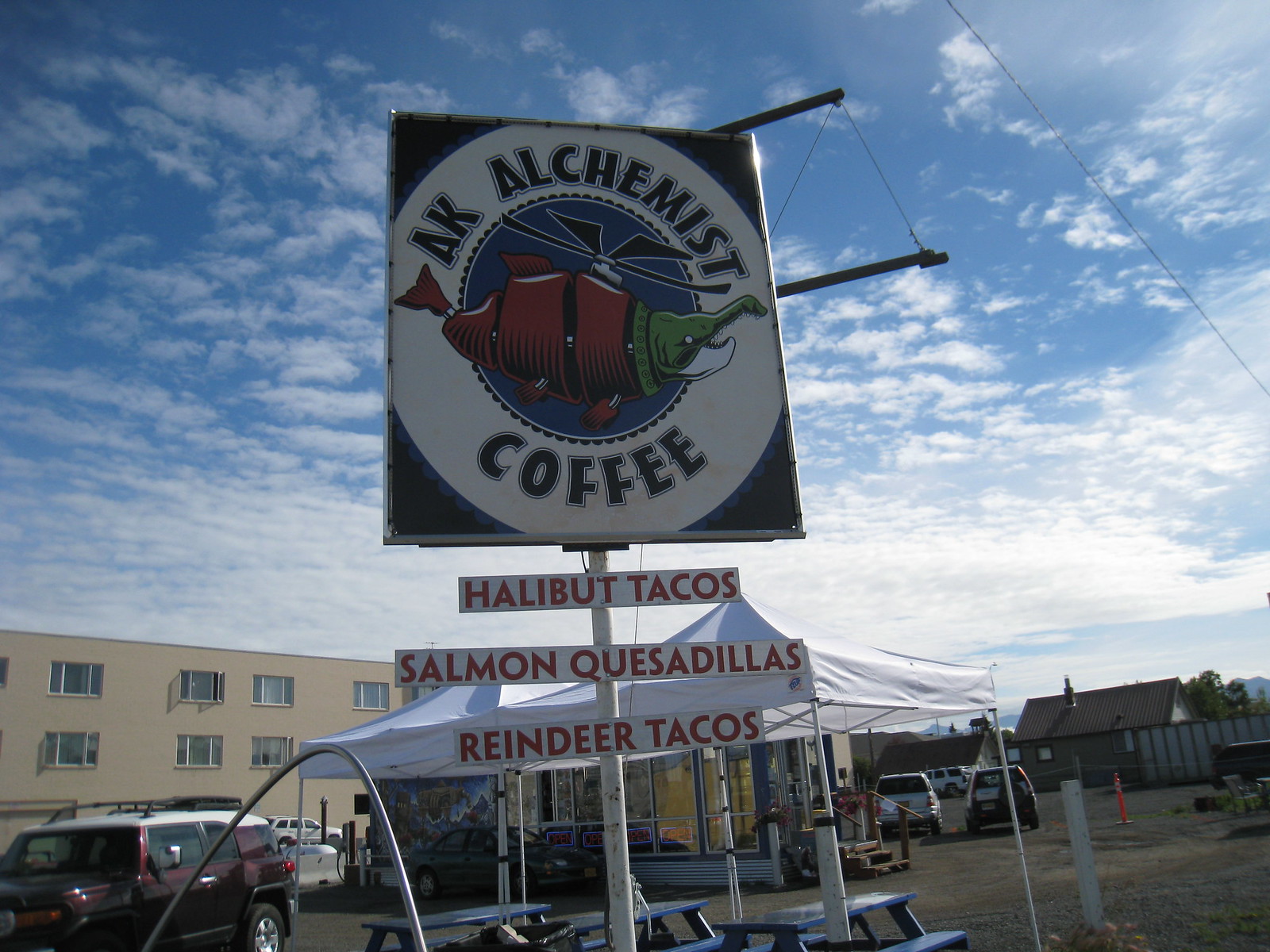The image depicts an outdoor street restaurant with a prominent sign on a large pole reaching into the blue sky, dotted with white, puffy clouds. The sign features a white circle with the text "AK Alchemist Coffee" in black around the edges. Inside the circle, there's a quirky image of a helicopter-themed hybrid creature with a fish body and crocodile head. Below the main sign, there are three smaller signs with white backgrounds and red lettering, advertising "Halibut Tacos," "Salmon Quesadillas," and "Reindeer Tacos." In the foreground, there's a white canopy shading blue picnic tables where patrons can sit. The restaurant itself is a small stand situated further back in the image, surrounded by a few parked cars. To the left of the scene, a large, beige, three-story apartment building is visible, adding to the urban atmosphere.